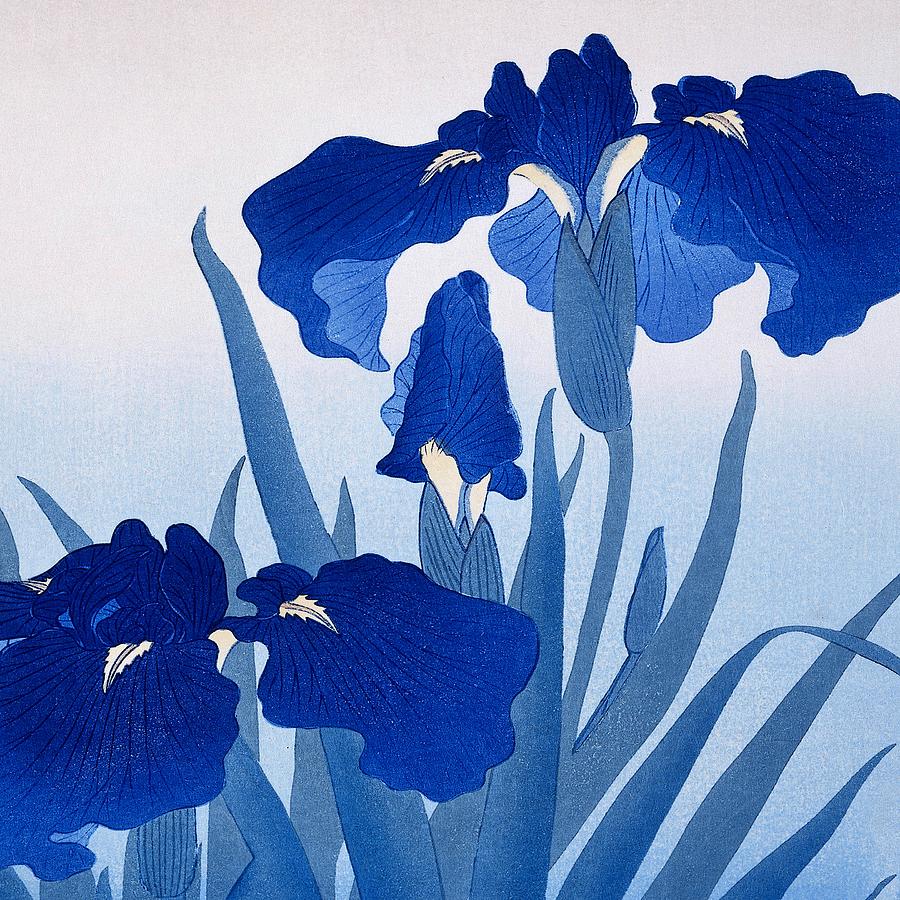This painting features an artistic portrayal of blue flowers and grasses set against a background that transitions from an off-white at the top to a deep blue gradient at the bottom. The flowers themselves, painted with watercolors, exhibit varying shades of blue. The fully bloomed flowers in the upper right have three distinct petals—a deep, dark blue with hints of white near their centers. 

The lighter blue reeds of grass contrast with the deeper blue hues of the flowers. The greenish-blue stems and parts of the plants add depth and variation. Detailed lines are drawn through the petals, adding texture and a sense of movement. The background incorporates nuanced color transitions, including light pink and green, blending smoothly into the blue gradient. Yellow and cream highlights punctuate the piece, emphasizing the dynamic composition. A tall flower occupies the center-right, while a smaller one is situated in the lower left, balancing the overall arrangement.